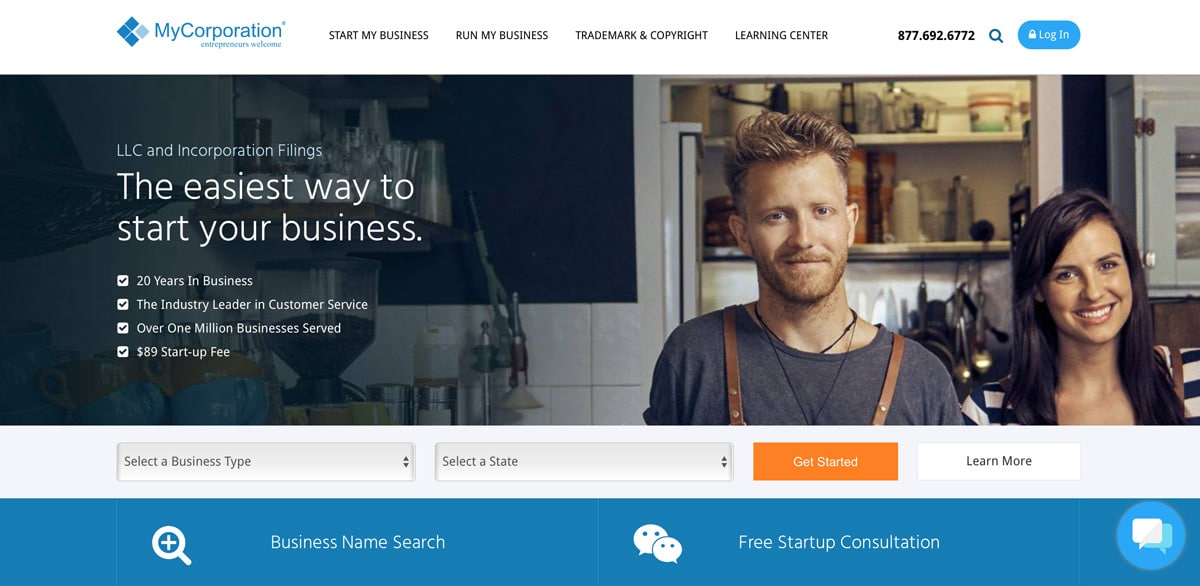Home Page of MyCorporation: 

The homepage of MyCorporation features a logo on the left-hand side with the company name, "MyCorporation," in one word. The logo consists of four squares, with one slightly misaligned and colored sky blue, contrasting against the blue of the other squares. 

Navigation tabs are prominently displayed across the top: "Start My Business," "Run My Business," "Trademark & Copyright," "Learning Center," and the customer service phone number 877.692.6772. To the right, there is a search icon followed by a blue login button. 

Below this header, an image showcases a friendly scene of a woman and a man in a kitchen. Both are wearing aprons over their t-shirts, embodying the look of casual, hardworking small business owners. Smiling, they stand in front of kitchen cupboards filled with dishes, utensils, and a coffee grinder, reinforcing the community-oriented, hands-on approach of many entrepreneurs.

Accompanying text reads: "LLC and incorporation filings - the easiest way to start your business." Below this tagline, there are vertical bullet points, each with checkmarks, highlighting the company's credentials: 
- 20 years in business
- The industry leader in customer service
- Over 1 million businesses served
- $89 startup fee

Beneath these points, users are prompted to "Select a Business Type" and "Select State" using drop-down arrows, with an orange "Get Started" button and a white "Learn More" button next to these selections.

At the bottom of the page, set against a blue background, further tools include a search icon followed by "Business Name Search," chat conversation bubbles, "Free Startup Consultation," and two interactive text boxes for user input.